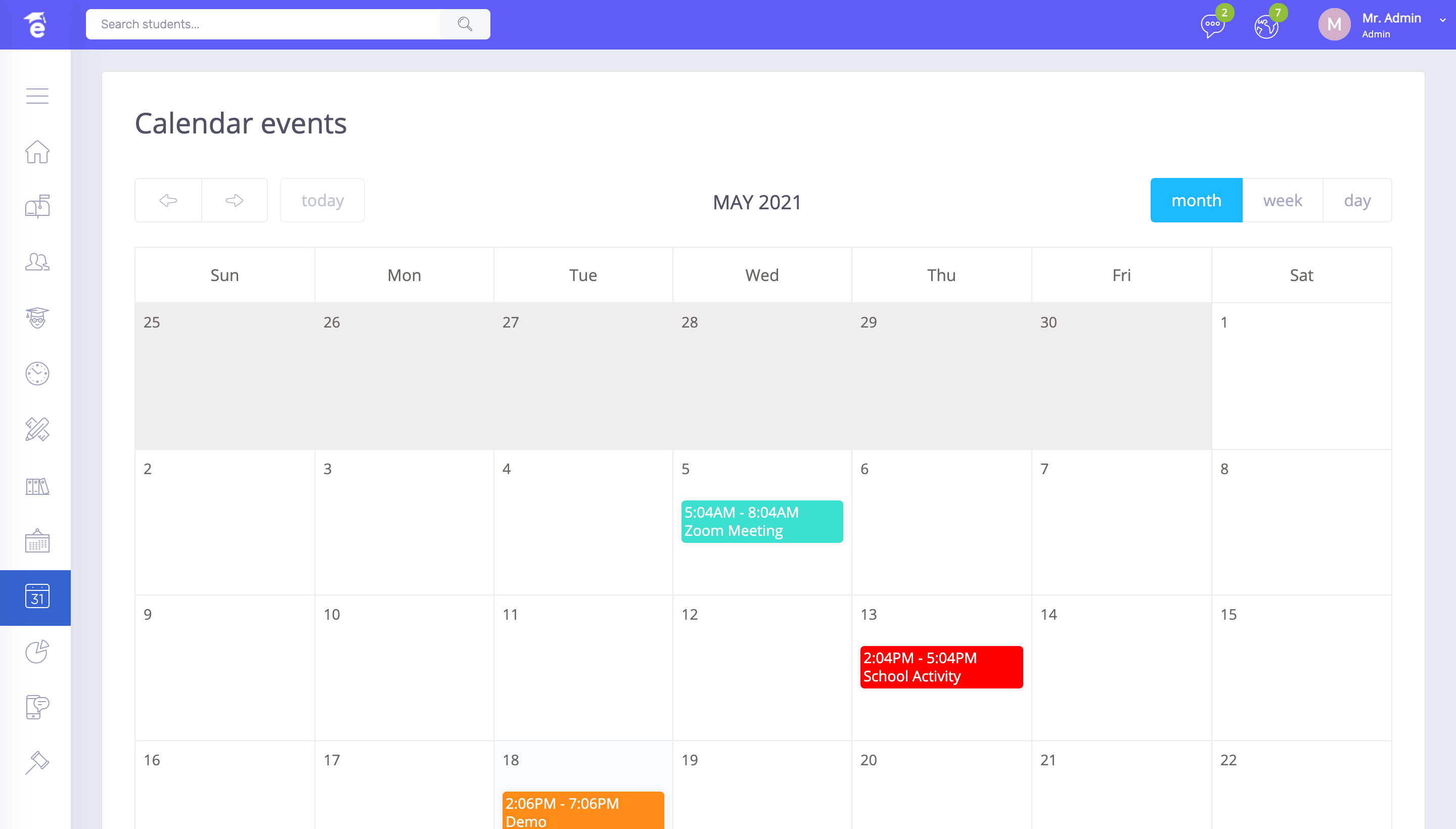The image showcases a website interface with a detailed and vibrant layout. At the top, there's a purple banner that resembles blue-violet but leans more towards purple. On the left side of the banner, there is a lowercase "e" adorned with a star resembling a graduation cap above it. Moving to the right, there is a search bar labeled "Search students..." accompanied by a magnifying glass icon at the end.

On the far right side of the banner, there's a thought bubble icon with small circles inside, topped by a green circle with the number "2." Next to it, there's a globe icon also topped by a green circle with the number "7." Adjacent to these, there is a light pink circle with a brown base containing the letter "M" and labeled "Mr. Admin," along with a drop-down menu indicating administrative options.

Below the banner, the left side features a vertical menu with various icons. In the center of the screen is a calendar section titled "Calendar Events." The calendar has navigation arrows to move to the previous or next time period and a “Today” button. The calendar displays the month "May 2021," with options to view the calendar by month, week, or day. Currently, the monthly view is selected, highlighted with a blue background.

The calendar grid shows abbreviated days of the week: Sun, Mon, Tue, Wed, Thu, Fri, and Sat. The top row is grayed out, indicating non-current dates. May 1st falls on a Saturday, and key dates include meetings on May 5th, a demo on May 18th, and a school activity planned for May 13th.